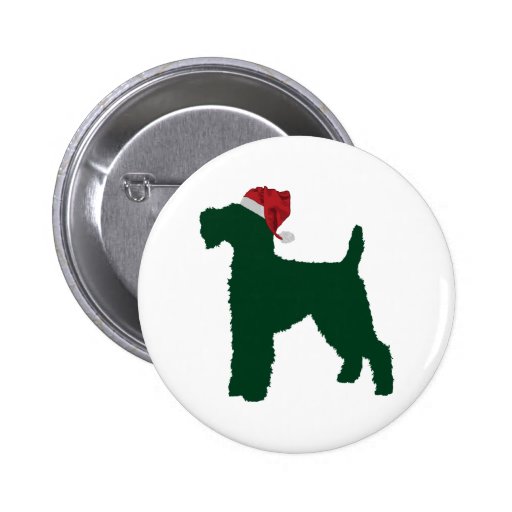The image depicts two circular pins typically worn during Christmas. The prominent pin in the front features a white background with the green silhouette of a medium-sized dog, possibly a Scotty Dog, Yorkshire Terrier, or Schnauzer, facing left. The dog is adorned with a detailed, realistic Santa hat—red with a white trim and a ball at the tip of the bent-down tassel. The dog has distinct features: a short, stumpy tail, four legs with the back legs spread apart, and a bushy area around its mouth. Behind and slightly above this pin, there's a partial view of another pin's backside, made of silver metal with a pie-shaped design. Visible is the clasp mechanism used to affix the pin to clothing.